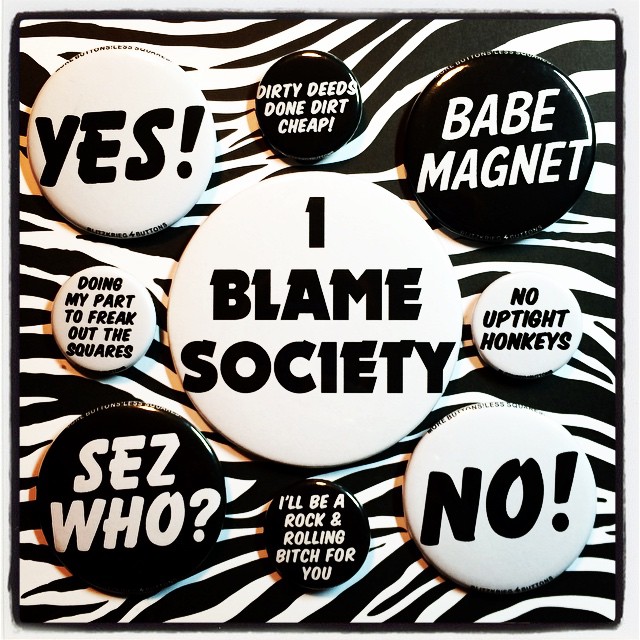The image is a striking black-and-white composition featuring a collection of circular metal pins arranged on a zebra-printed background. All the pins display text in either black font on a white background or white font on a black background. Shadows cast by the pins hint at yellow lighting from above. The collection includes a variety of provocative and whimsical messages. In the top left, a white pin announces "YES!" followed by a smaller black pin stating "Dirty Deeds Done Dirt Cheap." A larger black pin boldly declares "Babe Magnet." In the center, a smaller white pin reads "Doing My Part to Freak Out the Squares." A prominent white pin with black lettering says "I Blame Society." Another white pin, next in line, proclaims "No Uptight Honkies." Towards the bottom, a medium-sized black pin asks "Says Who?" and another declares "I'll Be a Rock and Rolling Bitch for You." Finally, a white pin simply says "No." The pins nearly cover the entire square mat beneath them, creating an eye-catching display of monochromatic design and expressive statements.